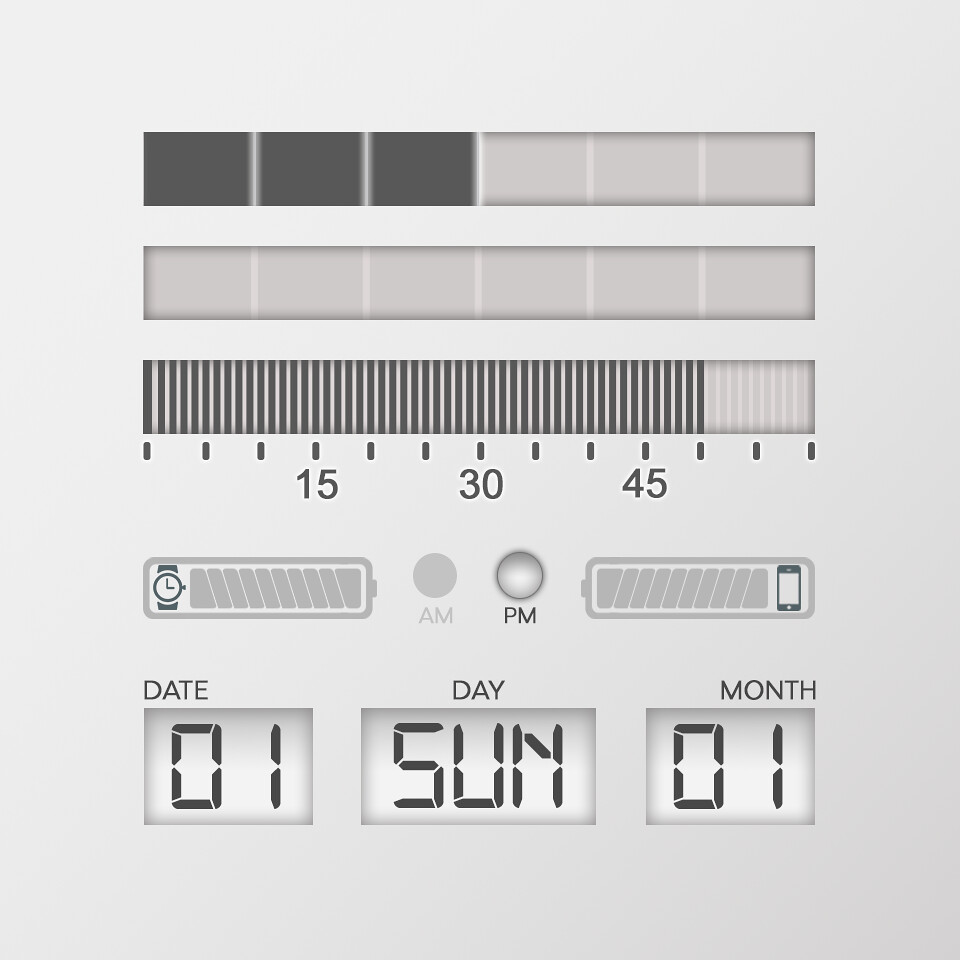The image showcases a digital-style clock with an intricate design. The primary feature is a set of horizontal bars, composed of 12 squares—six dark-colored squares on the left and six light-colored squares on the right. Beneath these, a series of light-colored squares are arranged together. Below, a numbered bar displays the markings 15, 30, and 45, with smaller incremental lines in between, extending slightly past the 45 mark with a dark indicator.

Additionally, there are two horizontal icons: one depicting a watch and the other a battery, indicating the time and battery status respectively. The display also includes "a.m." and "p.m." indicators, with "p.m." being illuminated. The date is shown as the first day of the month, with the day being Sunday and the month denoted as January. The entire display is set against a neutral gray background, creating a sleek and organized interface.